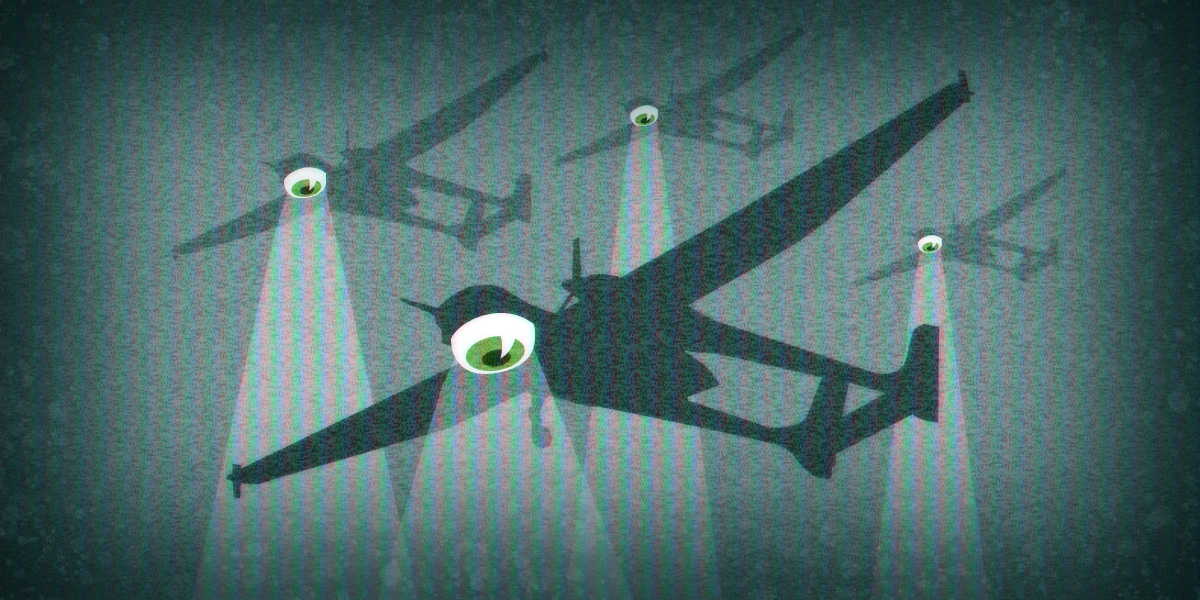The image is a detailed digital illustration with a greenish hue, depicting four unique drone-like planes flying in the sky. The background is a dark grayish-black with thin vertical red stripes subtly blending into the scene. The composition, viewed from the ground looking up, shows the drones concentrated in the central area of the horizontal image, positioned closer to the top. 

In the foreground, a larger, almost black drone dominates the scene, casting a substantial shadow. This foreground drone features a prominent green eye on its underside, projecting a bright spotlight toward the ground. Behind it, three smaller drones, shaded in more muted grays, also have green eyes on their undersides, each casting its own spotlight downward. These drones appear as shadowy silhouettes against the intricate background, adding depth and emphasis to the central theme of omnipresent surveillance.